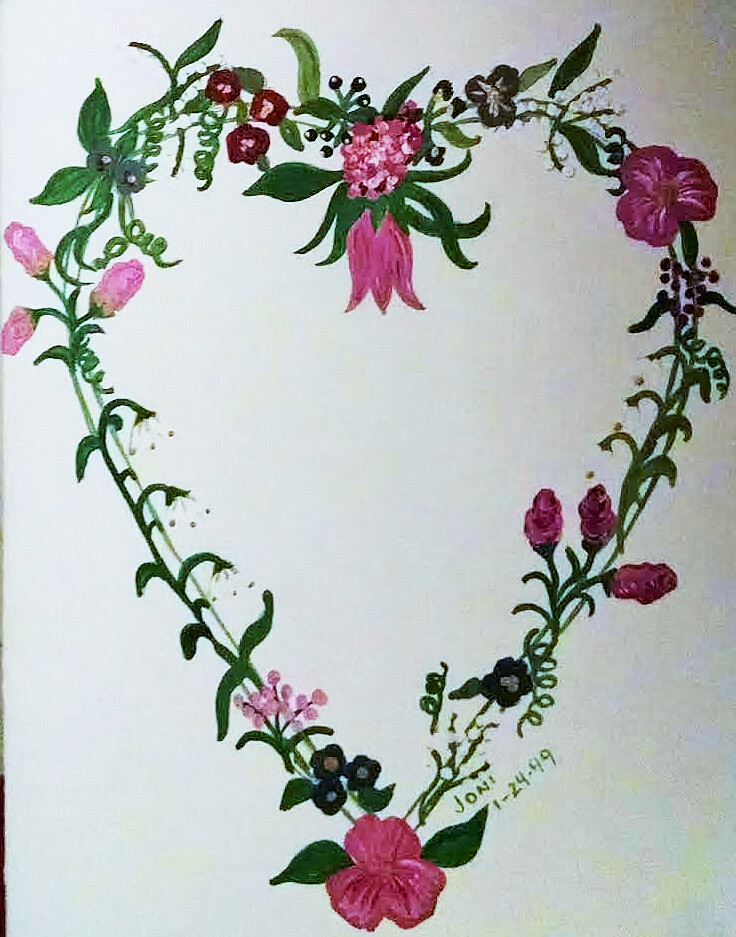This photograph captures a painting that showcases an intricately designed heart made from plant vines, set against a white background. The image quality is slightly grainy and darkens subtly on the right side. The bright green vines and leaves elegantly form the shape of a large heart that dominates the entire frame. Adorned with a variety of flowers, the heart features a spectrum of colors and shapes. At the bottom, a stunning pink flower stands out prominently. Ascending to the left, three small black flowers are positioned next to delicate pink-dotted blooms. Continuing upward, there are three white flowers followed by three pink ones. The top of the heart is graced with deep red flowers, and in the center lies an eye-catching, large pink flower. As our gaze moves to the right, another black flower is accompanied by more dotted white flowers, a pink flower, black-dotted flowers, three teacup-shaped white flowers, three pink flowers, and a tiny black flower succeeded by a white one. On the bottom right corner of the painting, the signature "Joni 124.99" is inscribed.